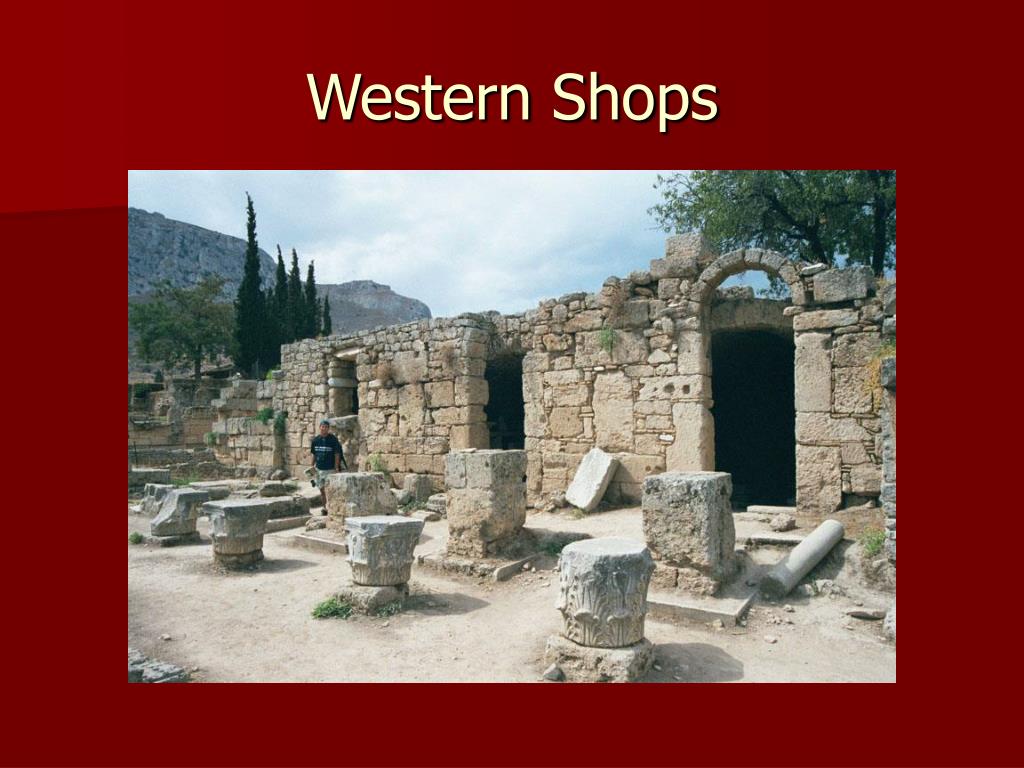This horizontal rectangular image appears to serve as an advertisement for an unspecified location. Dominated by a brownish maroon background, the image features prominently displayed yellow text at the top reading "Western Shops." Below the text, the central focus is a photograph of ancient ruins consisting of roofless stone walls and bases of pillars that have been worn away over time. The foreground is sparse, leading the eye toward the far background where a person stands in front of one of the dilapidated structures. The old stone ruins are framed by a mostly cloudy sky with patches of blue, and tall trees rise in the background. The overall composition, with the photograph situated toward the bottom and text at the top, resembles the layout of a presentation slide, perhaps akin to a PowerPoint slide. The color palette includes hues of brownish maroon, yellow, red, green, blue, gray, and white, adding to the visual richness of the scene.